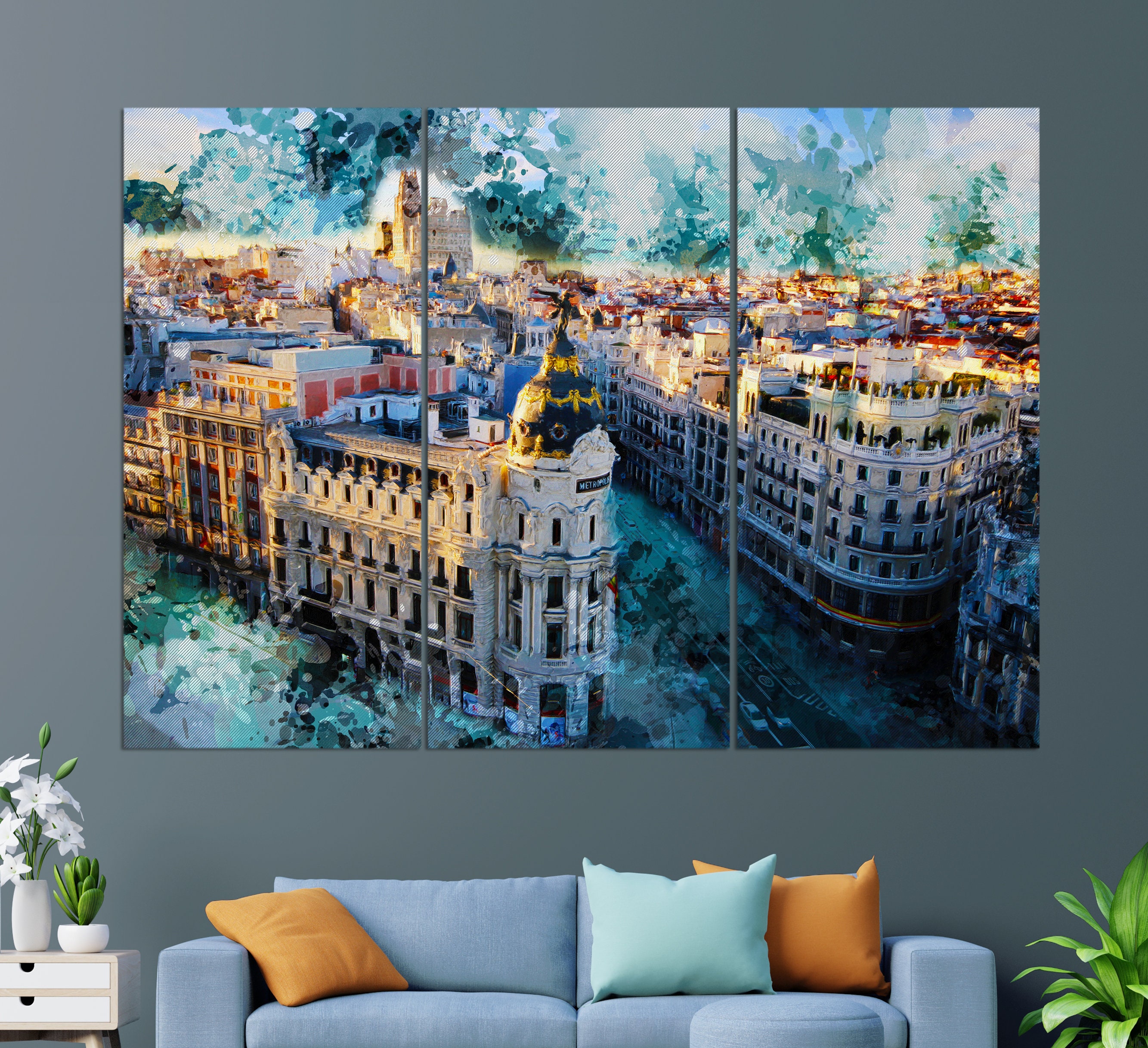The image showcases a modern-day living room with medium blue walls. Central to the decor are three canvases depicting an impressionist-style scene of a bustling European city, potentially featuring landmarks like Notre Dame, suggesting it could be Paris or another historic city. The buildings in the artwork are adorned in hues of gray, red, blue, gold, and green, with a roadway running between them and a dynamic sky painted with blues, greens, grays, and whites in the background. Below the artwork stands a light blue couch adorned with three pillows—two orange pillows flanking a light blue pillow. On either side of the couch are potted plants adding a touch of greenery to the setting. To the left of the couch is a small side table with two drawers, decorated with vases holding greenery and white flowers, contributing to the room’s elegant and vibrant aesthetic.